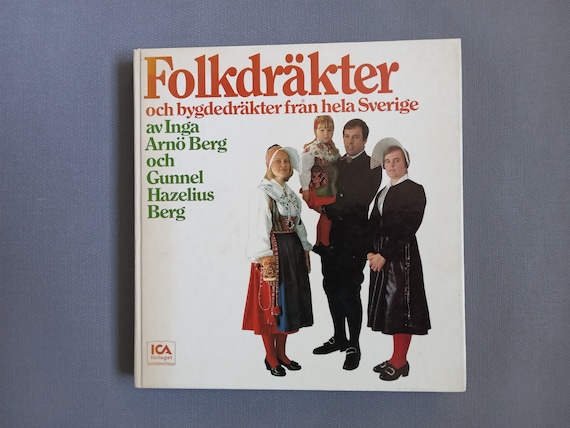The image depicts a color photo of a hardback book set on a gray table. The book cover is white and prominently features the title "Volk Dritter Ach" by Dietrich von Hitters Severage at the top. The lower left corner of the cover has the letters "ICA" in green. The centerpiece of the cover is a family of four, likely of European origin, dressed in traditional costume-like attire. 

The family includes a mother on the right, wearing a black sweater, black skirt, red stockings, black shoes with gold buckles, and a distinctive large white hat. Next to her is a father in a black jacket and pants, holding a small child. The man is also wearing black shoes. The child is dressed similarly to the older daughter, who is on the father's left. 

The older daughter is depicted in a blue and red skirt, with red stockings and black shoes. Her attire includes embroidery trim, adding to the ornate look of the family's costumes. The elaborate details and the traditional elements of their clothing suggest a cultural or festive theme, possibly from German, Dutch, or Ukrainian heritage.